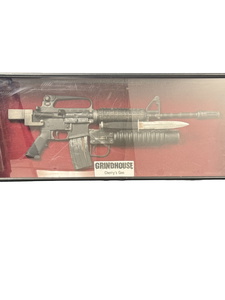The image depicts a steely gray assault-style weapon that seems to be a prop from the movie "Grindhouse," as indicated by a white label at the bottom of the display case. The weapon, encased in glass with a black border, rests on a red velvety material, accentuating its menacing appearance. The rifle, which lacks a stock, features a magazine protruding from the bottom and an underbarrel attachment. Notably, a knife or bayonet is affixed to the underbarrel, with silver accents on both the knife and the rear part of the weapon. The rifle also sports a double sight system, with sight positions near both the barrel and the back of the gun, adding to its detailed and combat-ready design. The reflective glass case securely protects the weapon, highlighting its display nature and making it resemble an exhibit, possibly in a museum or a similar curated setting.